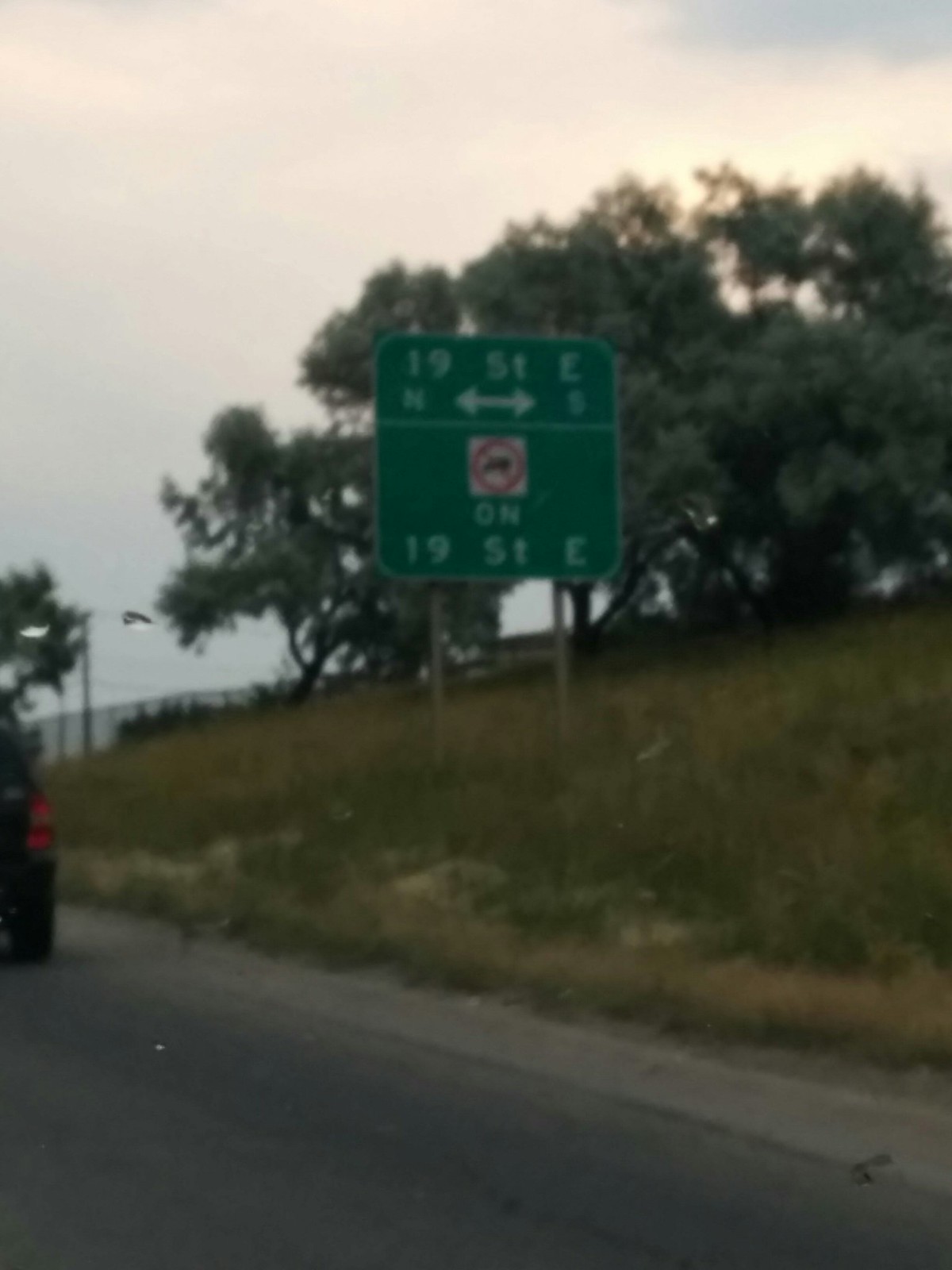The image captures a serene early morning scene beside a road, as indicated by the soft pinkish-blue sky suggesting the dawn hours. The gray asphalt road runs diagonally across the frame, leading the viewer's eye toward a hazy horizon. On the road, we can see parts of two vehicles: a truck and a dark-colored car, possibly dark red or dark gray, positioned ahead of the vantage point. 

To the right, a green grassy bank rises gently, forming a modest hill that adds a touch of natural beauty to the scene. In the distance, a fence lines the horizon, marking the boundary between the road and the cluster of trees dotting the background, adding depth to the image.

Prominently featured on the roadside is a green, squarish sign with rounded edges, mounted on two slender, silver poles. The sign displays "1951 East" at the top, accompanied by a double-headed arrow pointing in both directions. Below, the sign indicates "19th Street East" and includes a logo depicting a truck with a red circle and a red line through it, signaling a restriction on truck entry. The overall composition blends elements of nature and infrastructure, creating a quiet yet detailed roadside scene.